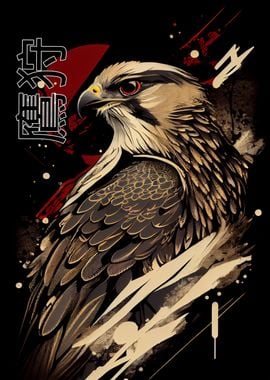This image portrays a detailed and stylized digital drawing of a proud hawk with a predominantly white head and gray feathers accentuated with hints of brown in its lower body. The hawk is depicted in a side profile with its body oriented to the right while its head is turned 180 degrees, gazing back over its shoulder. The hawk’s striking features include red eyes and a beak that is both gold and gray with a yellow tip.

Surrounding the bird is a black background punctuated by random splashes of red and white, adding a dynamic sense of movement to the composition. Additionally, white dots are splattered throughout, enhancing the overall visual texture. On the left-hand side of the image, there are two vertically written Asian symbols, possibly Korean or Chinese, filled in black with a white outline, contextualizing the piece with an Asian heritage. The amalgamation of distinct brush strokes around the hawk and the enigmatic symbols gives this artwork the impression of a poster or a scene from a graphic novel.